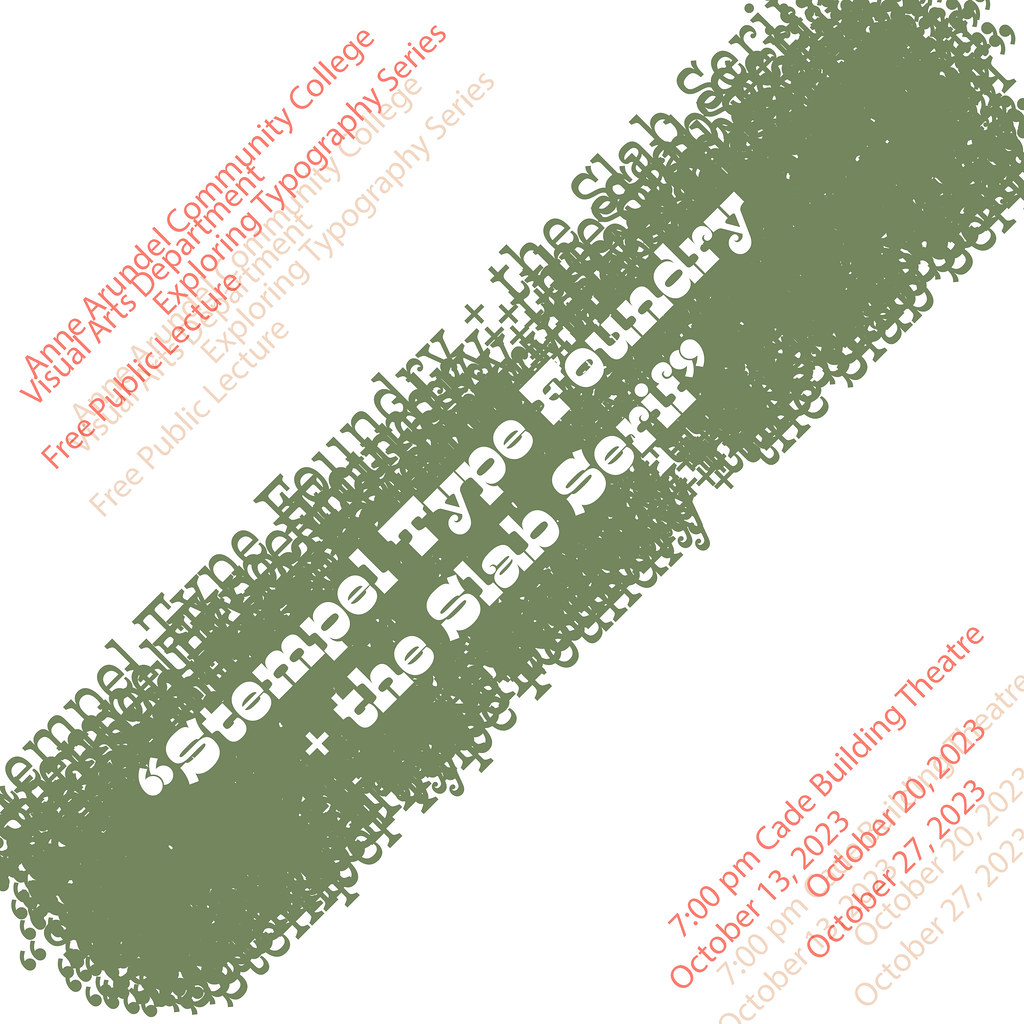The flyer features a creatively designed layout on a white background, with all text and elements arranged diagonally from the lower left to the upper center. At the top, written in pink/red ink, is the heading: "Anne Arundel Community College Visual Arts Department, Exploring Typography Series, Free Public Lecture." Below this, centrally located, is a green, capsule-shaped design filled with typography. The text within the green capsule alternates between green and white lettering, prominently displaying "MNL Tyne Foundry and the Slab Series," and "Stemple Type Foundry, The Slab Serif," the latter in quotation marks. Additional details in pink/red ink, also diagonal, highlight the event's schedule with three dates: October 13, 2023, October 20, 2023, and October 27, 2023, all at 7 p.m. at the Cade Building Theater. There are no images or artwork, emphasizing the typographic elements to create interest and excitement in the subject of typography.